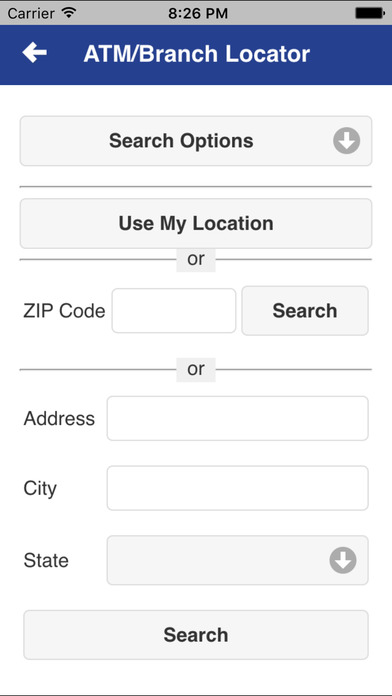This is a detailed screenshot of a mobile phone interface displaying an "ATM/Branch Locator" search feature. The interface is set against a white background. At the very top, there is a gray status bar showing various icons: on the left, the carrier name and a black Wi-Fi symbol, in the center, the time displayed as 8:26 p.m., and on the right, a black battery icon showing 100% charge. Directly beneath the status bar is a blue navigation bar with white text. Centered in the navigation bar is the title "ATM/Branch Locator," and to the left, there is a white arrow pointing to the left.

Below the blue bar are two selectable gray bars for search options. The first gray bar, labeled "Search Options," has a drop-down arrow on its right side, indicating additional choices are available. The second option is labeled "Use My Location." Underneath these options, users can manually input search criteria.

Three fields are provided for manual input: 
1. A white pill-shaped bar for entering the zip code.
2. Another white pill-shaped bar for entering an address at the top.
3. Below that, there is a white pill-shaped bar for the city, and finally, for the state, there is a drop-down arrow allowing selection from a list of states.

At the bottom of these input fields, there is a gray, pill-shaped "Search" button that users can click to initiate the search.